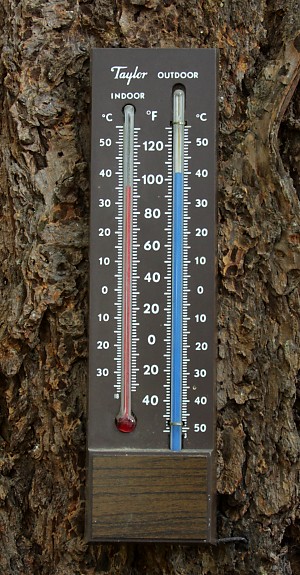In this high-quality image, we see a close-up photo of a dual thermometer, featuring both indoor and outdoor temperature readings. The thermometer, which appears to be mounted on either a table with intricate brown designs or possibly the oak bark of a tree, leaves its exact placement somewhat ambiguous due to the proximity of the shot. On the left-hand side of the device, a red fluid-filled tube marked "indoor" indicates a temperature around 100 degrees Fahrenheit (approximately 35 degrees Celsius). Adjacent to it, a blue fluid-filled tube labeled "outdoor" shows a reading of about 102 degrees Fahrenheit (around 40 degrees Celsius). The top left corner of the device is branded with the name "Taylor," and the thermometer's base is a rectangular piece of brown wood, providing a sturdy and classic foundation.